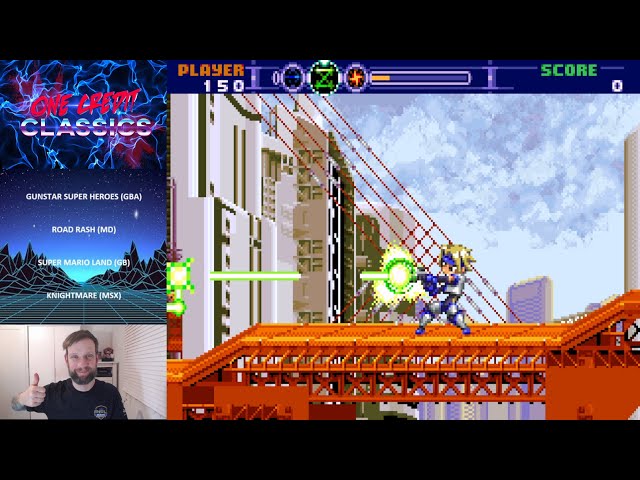The image is divided into four main sections, with the largest portion displaying a 1980s pixel sprite-style video game. The game features a blonde-haired character in silver and purple armor, firing a green laser beam to the left while standing on a golden-brown bridge. Behind the character are gray buildings against a grayish-blue sky. The game interface shows "Score: 0" in the top right and "Player: 150" along with various icons and a bar in the top left. 

In the top-left subdivision of the image, colorful text on a blue background reads "One Credit Classics." Directly below this section is a collection of screenshots labeled "Gunstar Superheroes GBA," "Road Rash MD," "Super Mario Land GB," and "Nightmare MSX," featuring a blue sky and black pixelated mountains. Beneath these screenshots is a photograph of a man wearing a black t-shirt, giving a thumbs-up.

The overall composition includes additional black bars at the top and bottom, giving it a widescreen appearance. The detailed blend of retro gaming elements and the inclusion of a participant's image suggests an engaging presentation centered around classic video games.